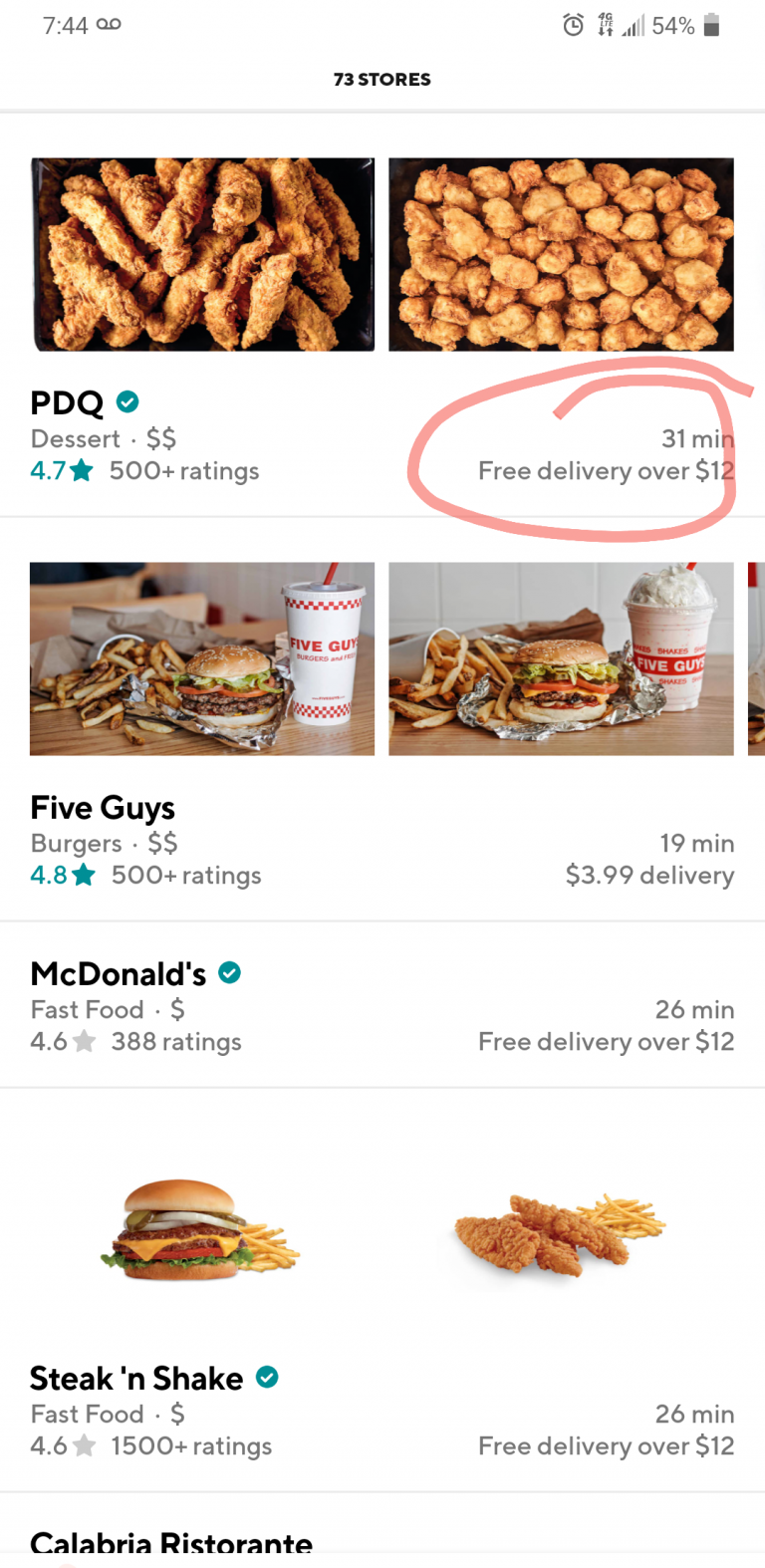The image showcases a cell phone screen featuring a food delivery app interface. In the top left corner, the time is displayed as 7:44, while the top right corner includes various icons such as an alarm clock and a battery indicator. Below these icons, it indicates that there are 73 stores available.

The main section of the screen is occupied by images of food items from different restaurants. On the left side, there is an image of a plate of chicken, and to the right, another image shows smaller pieces of chicken. Beneath these images, it reads "PDQ" accompanied by a blue circle with a white checkmark. The description next to it summarizes the offering: "Dessert, 4.7 stars, 500+ ratings." To the right, it states "31 minutes, free delivery over $12," and there is a red circle hand-drawn around this delivery information.

Further down, two more side-by-side images appear. The left image features fries and a hamburger accompanied by a cup labeled "Five Guys." The adjacent right image mirrors the contents but includes what seems to be a cup of ice cream. Above these images, the name "Five Guys" is mentioned along with the description: "Burgers, 4.8 stars, 500+ ratings," and delivery details: "19 minutes, $3.99 delivery."

Below this section, the screen lists "McDonald's" with a summary: "Fast food, 4.6 stars, 388 reviews," and states: "26 minutes, free delivery over $12."

At the bottom, there are two more images; the left side depicts a hamburger and fries, while the right side shows pieces of chicken and fries. Underneath, it reads "Steak 'n Shake," followed by "26 minutes, free delivery over $12."

Overall, the screen is a detailed interface of various food options available for delivery, complete with ratings, estimated delivery times, and delivery fee information.